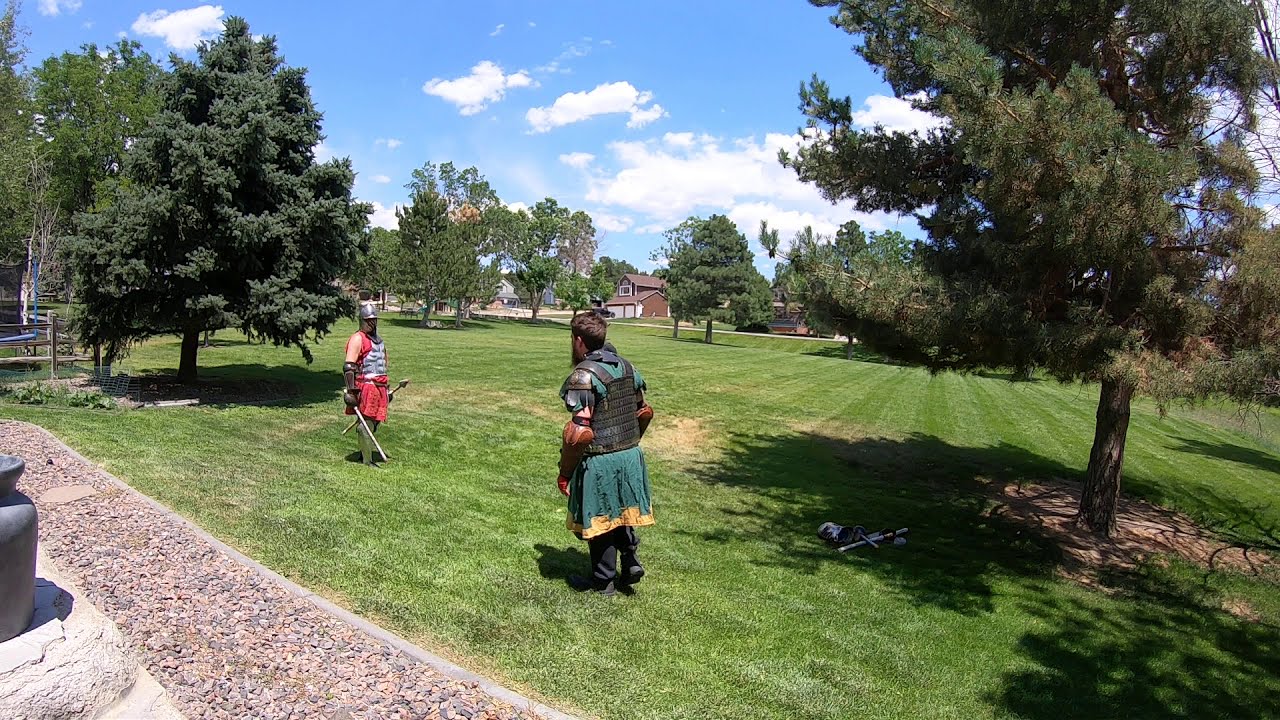This outdoor photograph captures a vivid reenactment of a medieval knights' duel set in a modern-day park. The scene centers on two men dressed in period-specific armor, poised as if about to engage in battle. The man on the left, dressed in a red tunic with grey accents and a metal helmet, clutches a sword while facing the camera. Opposite him stands another man in a green tunic with a gold-trimmed bottom and leather forearm guards, his back to the camera, with his sword lying on the ground beside him.

The grassy park is dotted with various trees, including pine trees, and appears around noon given the shadows fall directly beneath the trees. A house and some other modern elements are visible in the background, juxtaposing the historical costumes. Nearby, under one of the trees, lies a pile of various items, potentially more medieval equipment. The scene is framed by a blue sky with scattered white clouds, adding to the timeless feel of this vivid tableau of medieval role-playing.